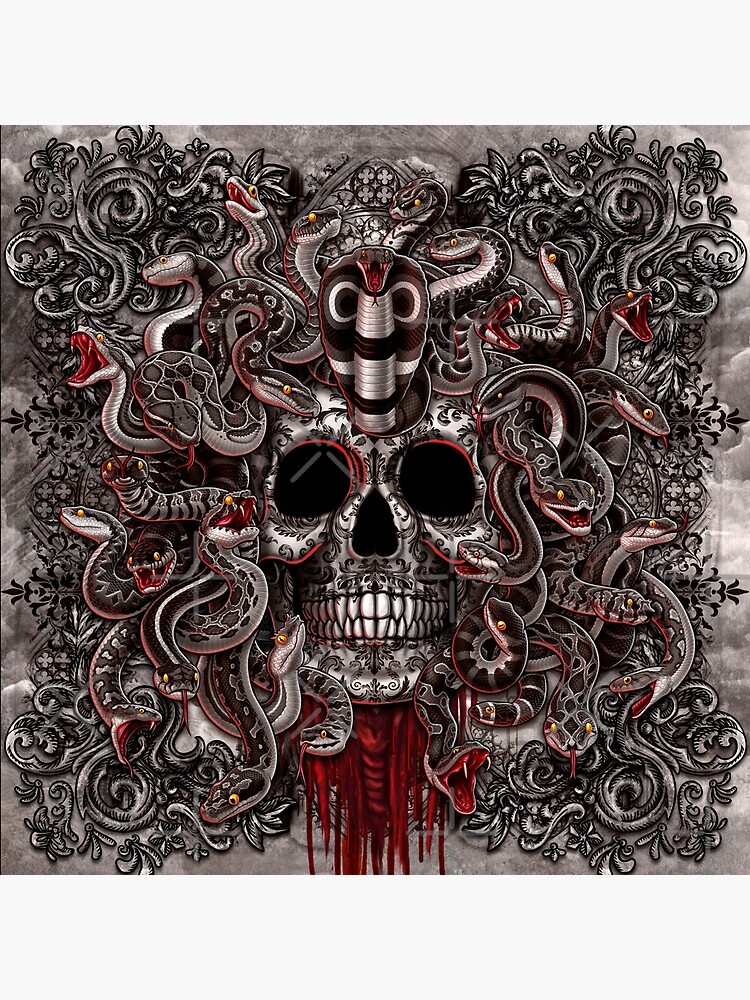The image depicts a highly intricate, computer-generated design set against a gray backdrop resembling cloudy shading. Dominating the scene is a metallic silver skull, etched with elaborate, black floral patterns. The skull's eyes are dark and hollow, its teeth stark white, resembling fangs. Around and emanating from the skull, multiple snakes with red outlines hiss menacingly, their mouths agape. The most prominent snake, a cobra with an extended hood, sits atop the forehead, its tongue protruding. Blood appears to drip from the base of the skull, creating a messy, red cascade down to where a spine might begin. The entire image is framed with black swirling designs that complement the ornate patterns on the skull, enhancing the dark, heavy metal aesthetic of the piece.